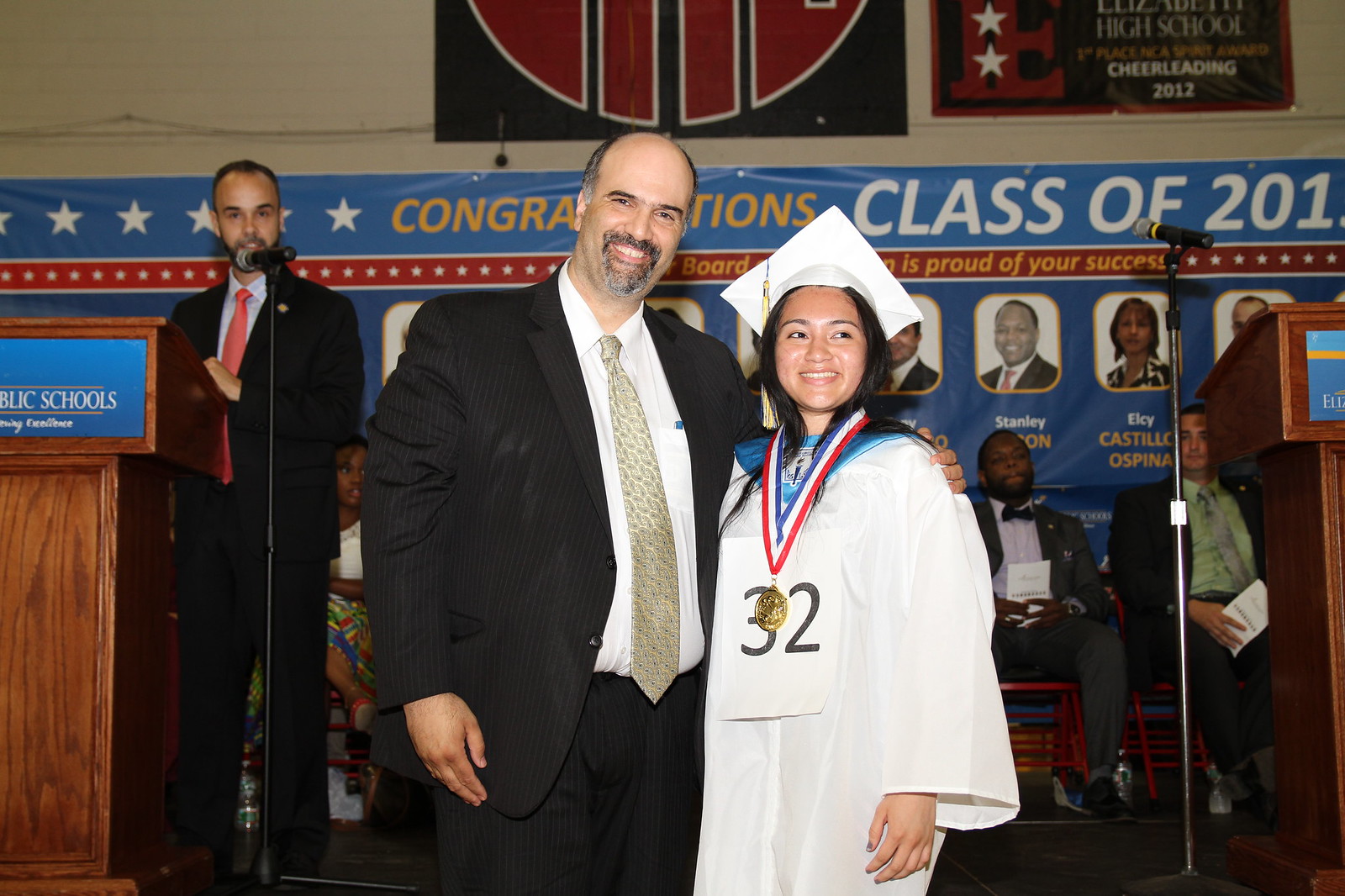The image captures the joyous moment of a high school graduation ceremony, set against a beige concrete block wall adorned with pictures of past graduates. Dominating the center is an older, light-skinned man with balding hair, a grayish beard, and a mustache. He is dressed in a black pinstripe suit, an unbuttoned white collared shirt, and a speckled beige or gold tie. Radiating happiness, he has a big toothy smile and his arm affectionately around a young Asian woman beside him. She is the focal point in her pristine white cap and gown, adorned with a gold medal on a red, white, and blue ribbon, and the number 32 on her chest. Both are smiling warmly at the camera. 

To the right of them, the blue background banner displays the partially visible message "Congratulations Class of 20xx," indicating the class year. The setting appears to be a school auditorium with a dais platform to the left, where another man stands behind a microphone. This man, too, has balding hair, a mustache, and a beard, and is dressed in a dark suit with a white shirt and a reddish-tinged tie. The scene is filled with various colors, but blue and white dominate, emphasizing the celebratory atmosphere of the graduation ceremony.